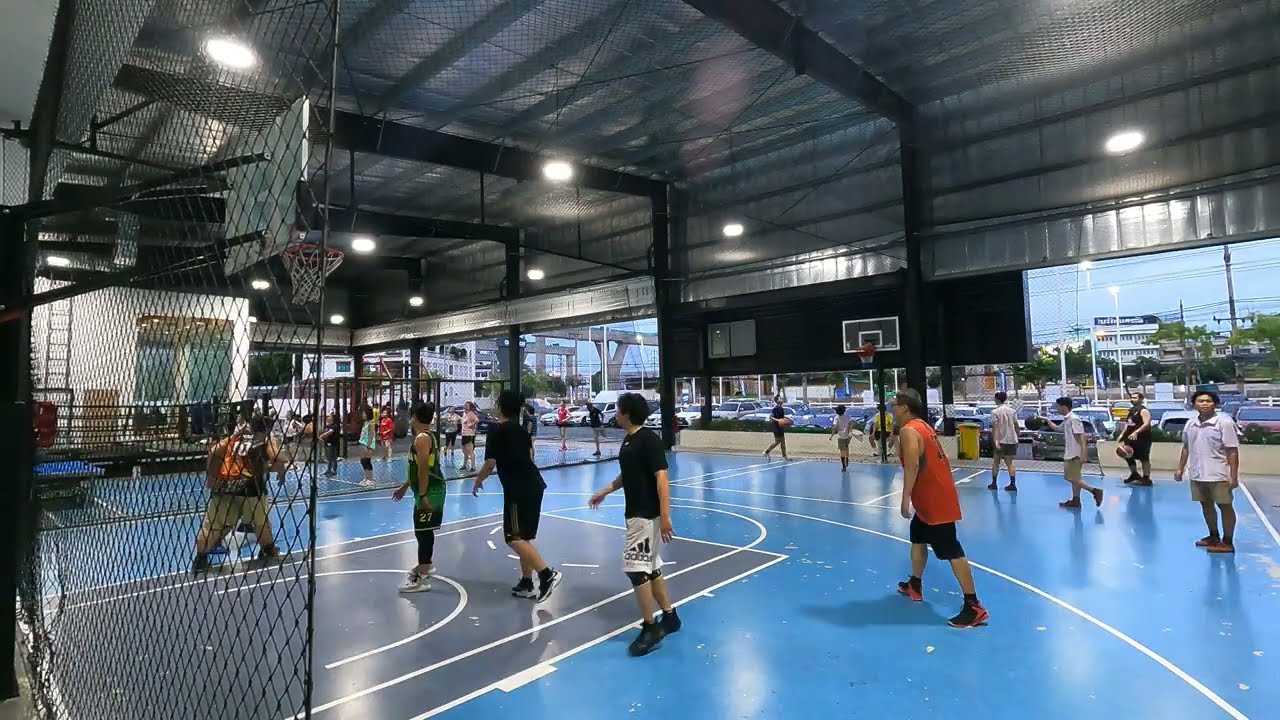This image depicts a semi-indoor basketball hall featuring a vibrant aqua blue court with crisp white lines, extending into multiple playing sections. The area is filled with a diverse group of individuals, mainly older kids and teenagers, actively engaged in basketball or gathering around the court, dressed in various sports outfits including sleeveless jerseys, sports shorts, and colorful sneakers. The court is enclosed by a black wire fence behind the clear-backboard basketball hoops, designed to prevent balls from escaping the play area. Overhead, the metallic silver ceiling, supported by black pillars and beams, is equipped with hanging lights. The far wall is open, offering a view of a cityscape adorned with a bridge or large overpass and a vast parking lot filled with numerous cars, blending the dynamic indoor activity with the bustling urban life outside.